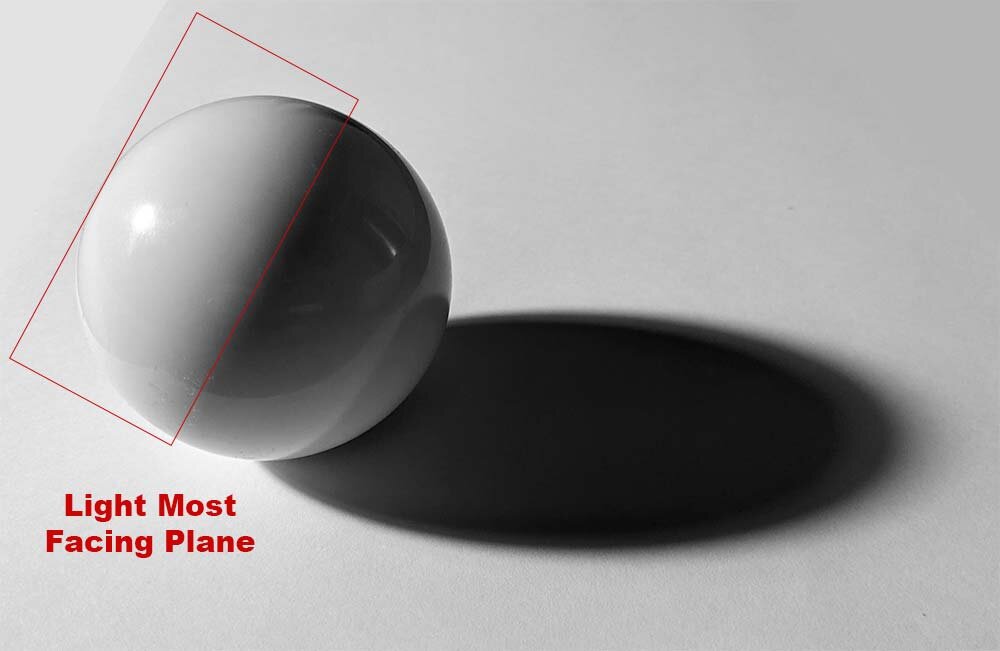The image features a photograph of a white spherical object, resembling a cue ball from billiards, positioned on the mid-left side of a light gray background. The ball is partially illuminated by an off-frame light source on the left, creating a distinct shadow extending to the right. The sphere's surface is divided by a red, thin-lined rectangular outline, slanted and positioned on the half facing the light source. This red rectangle highlights the illuminated portion of the sphere, reflecting its position relative to the light. Just below the sphere, bold red sans serif text reads "light most facing plane." The image appears to be a monochromatic photograph, with the exception of the red rectangle and text, and is likely used to illustrate principles of lighting and shadow in contexts such as mathematics or science.